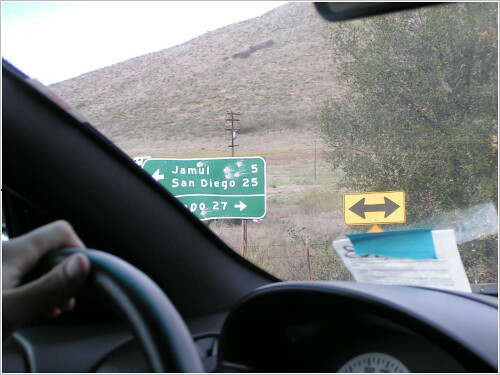The color photograph captures the view from inside a vehicle, focusing on the scene beyond the windshield. The image is taken from the driver's perspective, with a left hand visible on the steering wheel, and part of the dashboard and speedometer partially obscuring the windscreen. Through the windshield, several road signs are visible: a green highway sign indicating "Jamul" to the left in 5 miles, and "San Diego" straight ahead in 25 miles. There's also a yellow sign showing arrows pointing both left and right. The background features a steep, barren scrubland hill with sparse tufts of green vegetation, highlighted by an overexposed sky that appears almost white with a faint hint of blue in the top left corner. An additional detail is a sign or permit taped to the windshield, contributing to the sense of realism in the scene.